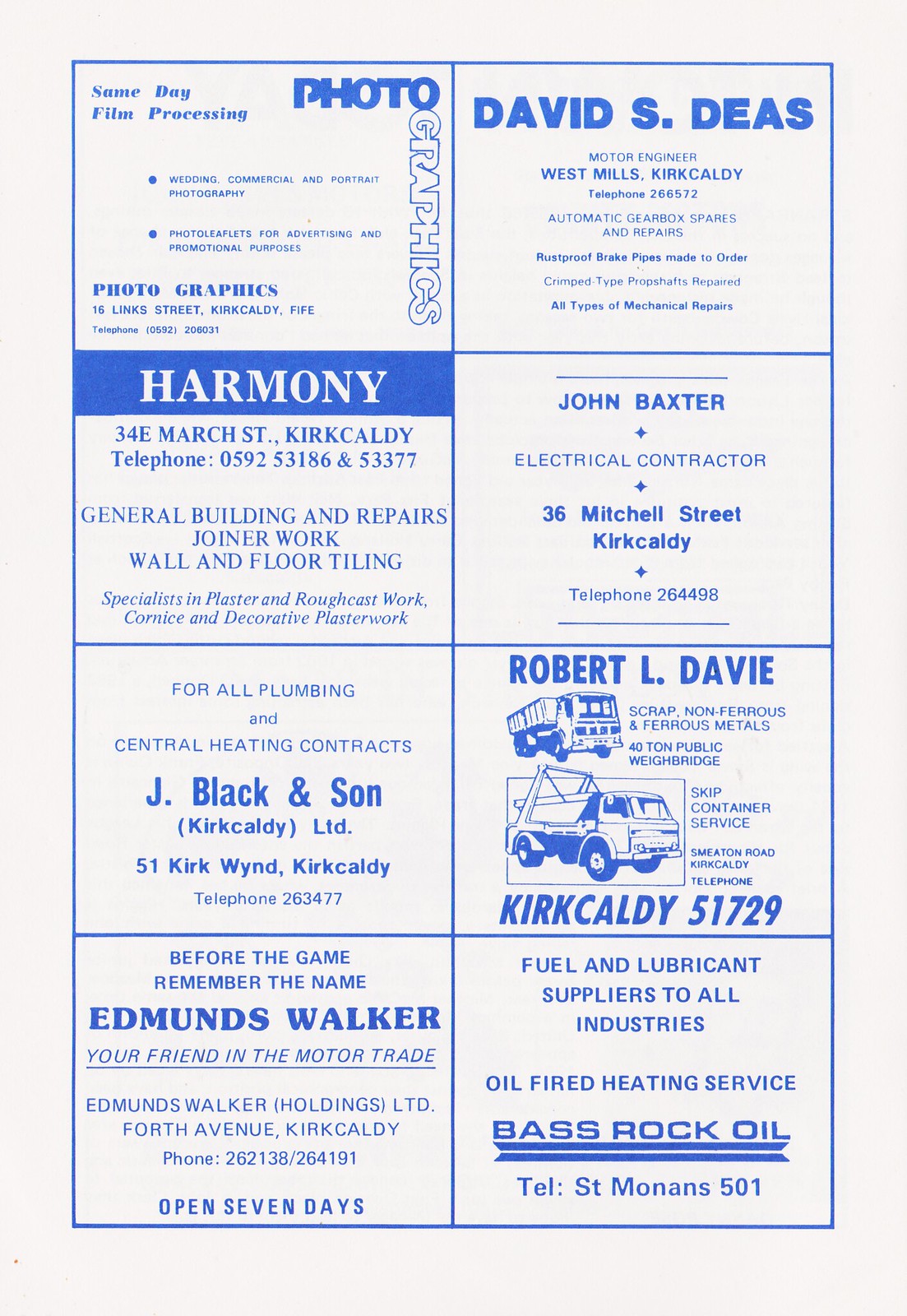The image depicts a page from what appears to be either a magazine or a game day program, primarily consisting of local business advertisements arranged in two columns of four ads each, set against a white background with blue text. 

Starting from the top left, the first advertisement is for "Photo Graphics," offering same-day film processing, wedding, commercial, and portrait photography, as well as promotional photo leaflets. Directly below, "Harmony" advertises general building and repair services, including joiner work, wall and floor tiling, and specialized plaster work. The third ad down in this column is "Jay Black & Son," which handles plumbing and central heating contracts. At the bottom left, "Edmunds Walker" promotes its services in the motor trade.

In the adjacent right column, the top ad features "David S. Dees," a motor engineer based in Wes Mills, Kirkcaldy. Below that is “John Baxter,” an electrical contractor located on Mitchell Street, Kirkcaldy. The third ad down in this column is for "Robert L. Davie," detailing services in scrap metal dealing and skip container service. Finally, at the bottom right, "Bass Rock Oil" advertises itself as a supplier of fuel and lubricants to various industries, also offering oil-fired heating services.

The overall style and setting resemble a page directly out of a book or magazine, with the page taking up the entirety of the image and showcasing an assortment of services provided by local businesses.